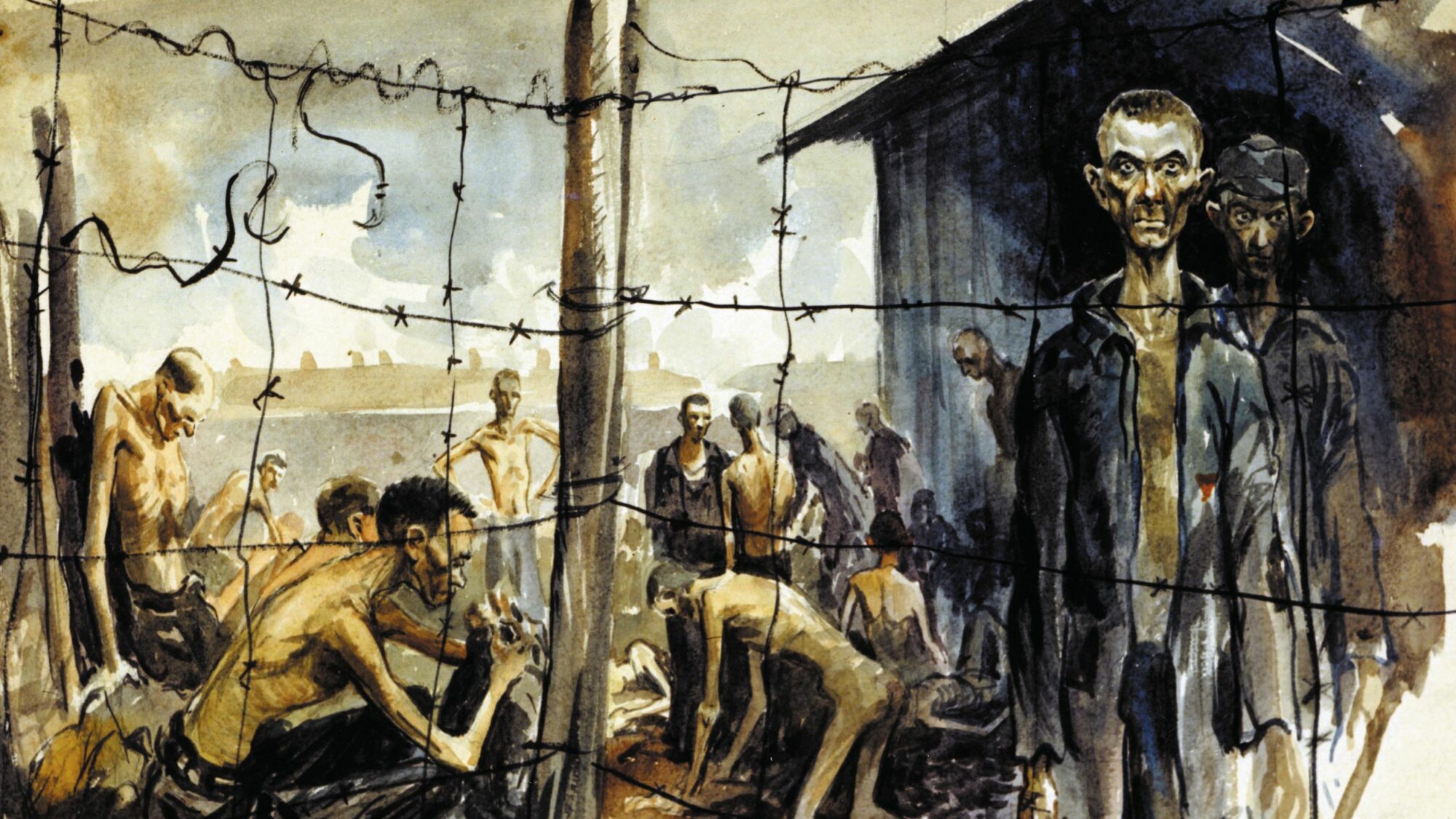This watercolour painting depicts a harrowing scene of men imprisoned in a camp, likely a concentration or POW camp. The men are standing behind a rudimentary barbed wire fence, supported by simple wooden posts. The background is overshadowed by a smoky, brown and blue sky, adding to the overall sense of desolation. The figures are emaciated, many with shaved heads and bony limbs. Some are barely clothed, with a few even naked. Those who are clothed mostly wear dark pants without shirts, exuding exhaustion and sickness. 

On the right side, two distinct men, one wearing a hat and the other with an unbuttoned shirt, stare directly at the viewer, their expressionless faces and prominent ears offering no solace. On the left, men are seen lounging, sitting, or tending to an individual on the ground, embodying a mix of despair and monotonous suffering. The color palette of grey, brown, and dark blue intensifies the bleak atmosphere, reflecting the sadness and despair that pierces through the melancholic scene.